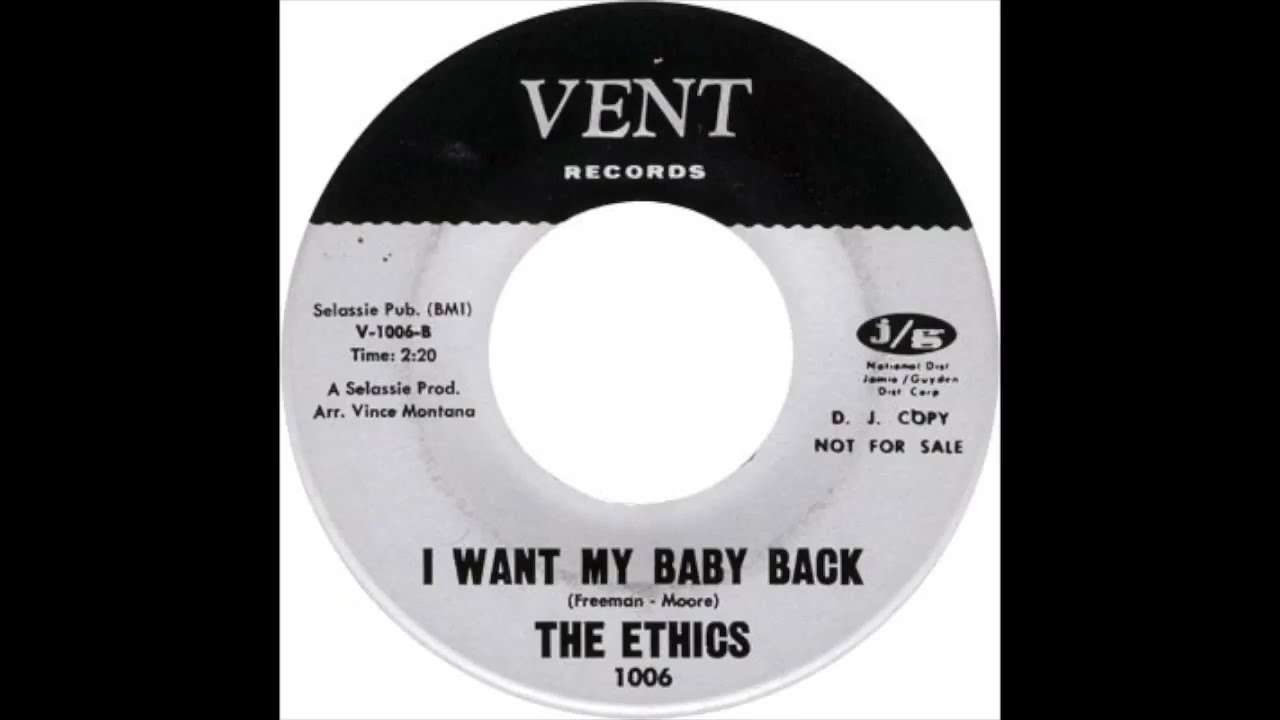The image depicts a black-and-white photograph of a circular vinyl record with a white background. The record, produced by Vent Records, prominently displays the title "I Want My Baby Back" by Friedman and Moore, performed by the band The Ethics. The label features several informative text elements: along the top it reads "Vent Records," and underneath, in light gray, is the text "Selassie Pub BMI V-106-8 time 2 minutes and 20 seconds, A Selassie Productions arranged by Vince Montana." To the right, a logo marked "J/D" is present with some smaller indiscernible text beneath it, followed by "DJ copy not for sale." The record’s catalog number, 1006, appears just below the band name. The image overall is stark, utilizing a grayscale color palette that emphasizes its vintage nature, capturing the feel of an old record archived, possibly digitized from a scan to preserve its details.